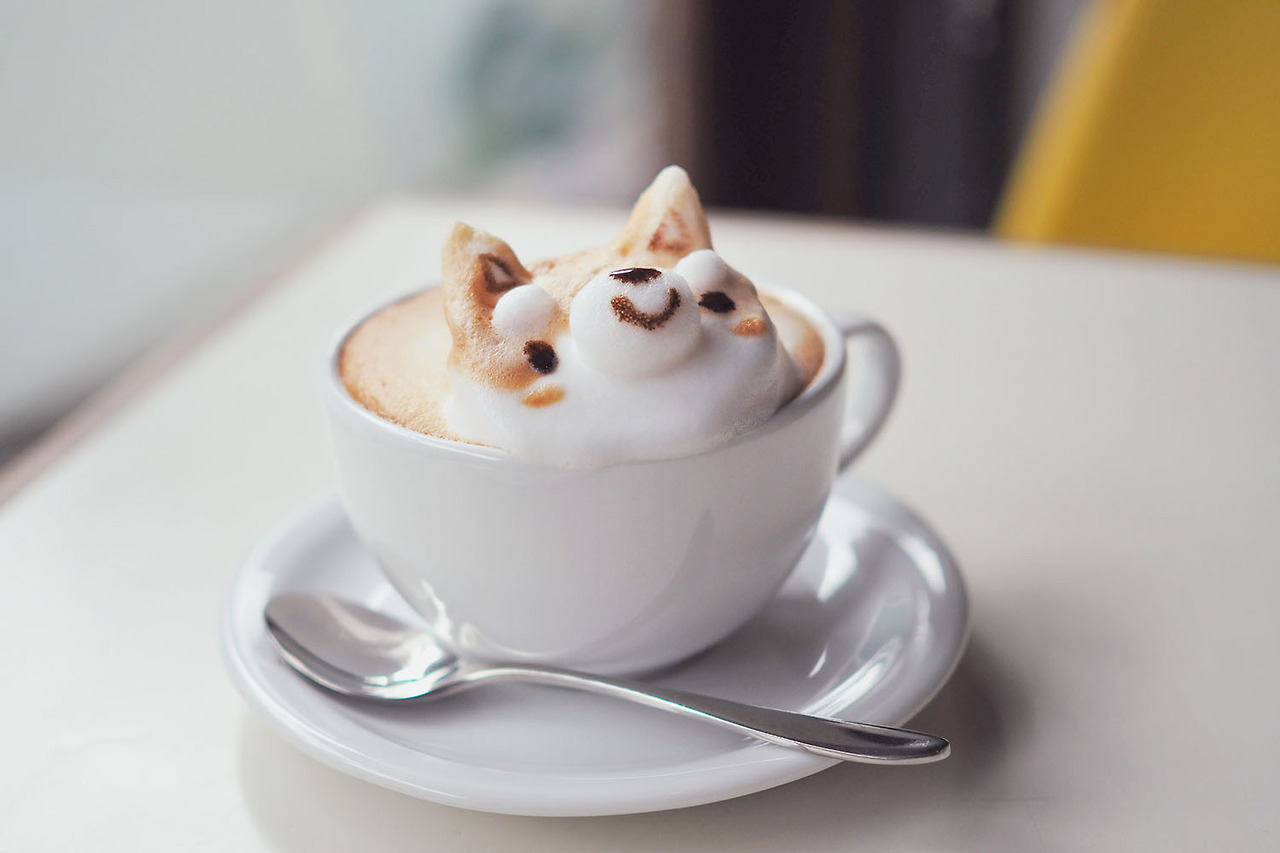In this professional photo taken at a cafe or coffee shop, a charming cappuccino cup is the focus. The white cup, with its slightly out-of-focus handle visible on the right, sits on a matching white saucer. A small silver spoon rests on the saucer, angled with the top facing away. The setup is placed on a white table, and part of a yellow, indistinct blur in the background—possibly a chair or an outfit—adds a touch of color. The coffee features intricate foam art, showcasing a dog with perky ears, a smiling face, and detailed eyes and nose crafted from brown and white foam. This whimsical creation brings the scene to life, set against a backdrop that suggests a cozy, street-side cafe ambiance.